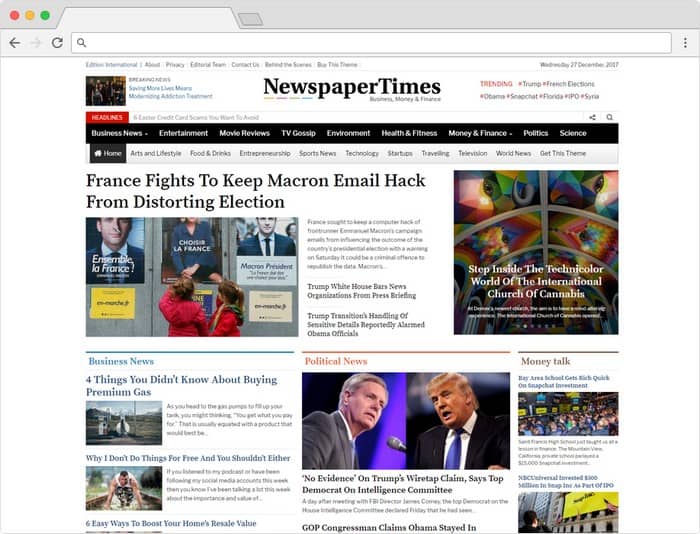This image is a screenshot from a web page. The top of the web page has a gray border, featuring three circles on the top left in red, orange, and green. Beneath those circles, there's a refresh button on the left and a back button. The address bar is empty. 

Directly below, "Newspaper Times" is prominently displayed in bold, black letters.

A black header bar beneath the title lists various sections: Business, News, Entertainment, Movie Review, TV Gossip, Embarrassment, Health and Fitness, Money and Finance, Politics and Science.

The main content follows, with a headline that reads, "French fight to keep Macron email hack from distorting the election." Below this headline is an image of people observing a poster of the President of France.

Further down, the page shows a picture of a man in a suit standing next to Donald Trump. To the left, there are article titles that include, "Four things you didn't know about buying premium gas", "Why I don't do things for free and you shouldn't either", and "No evidence on Trump's wiretap claims says top Democrat on intelligence committee."